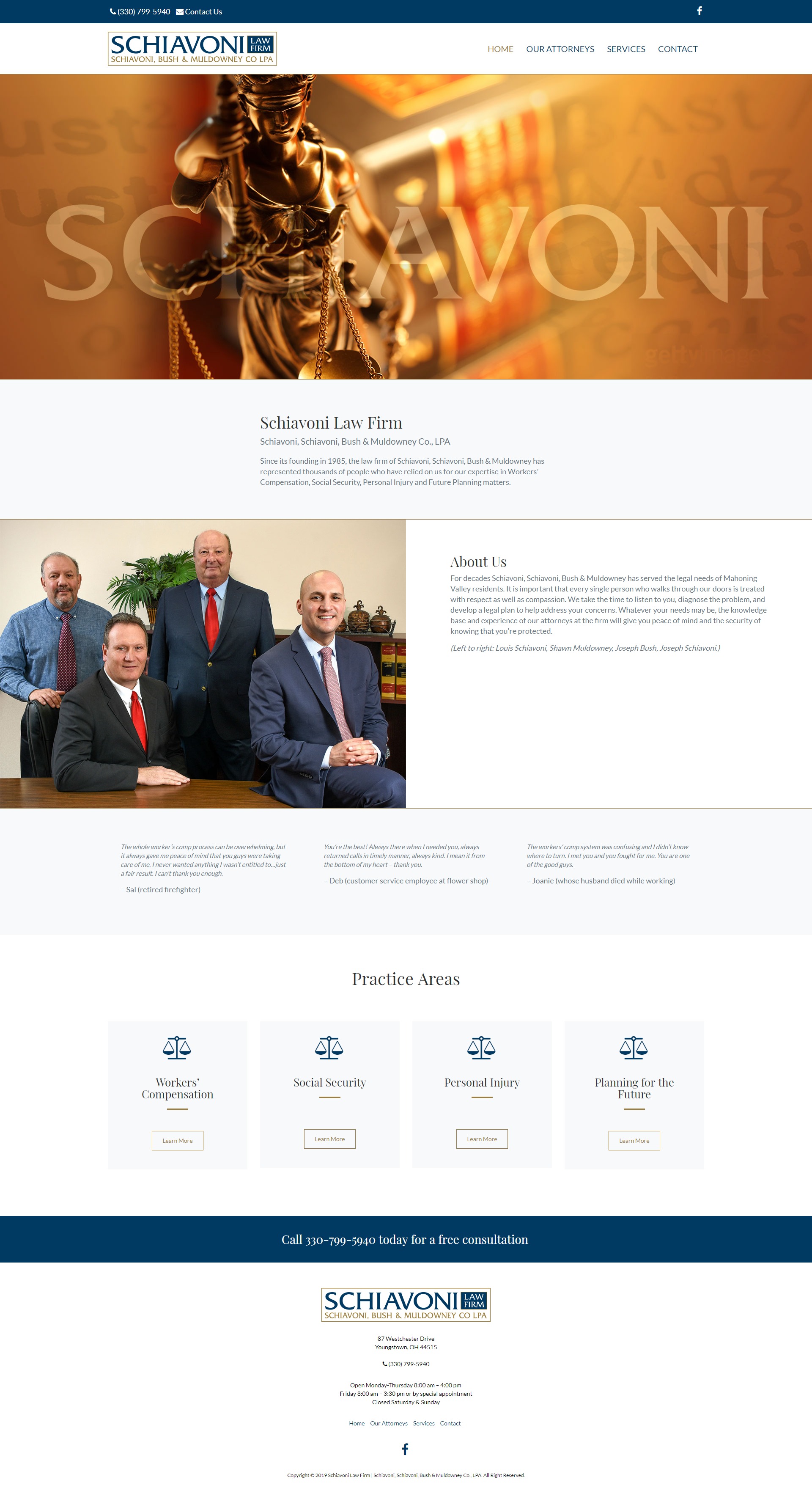This image appears to be a web page from the Schiavone Law Firm. At the top of the page, there is a gold-colored logo featuring a golden statue with the name "Schiavone" displayed prominently across it. Directly beneath the logo is a small section of print that is too small to read clearly.

Below the logo and text, there is a small photograph showing four men who seem to be the key figures of the firm, possibly the founders or directors. Three of the men are dressed in formal suits, while the fourth is in his shirt sleeves. Next to the photograph, there is a tiny label that likely reads "About Us."

The lower section of the page is divided into three text sections, each containing small print. These sections are likely descriptions of the firm's values, mission, and other foundational information, though the headings are also very small and difficult to decipher.